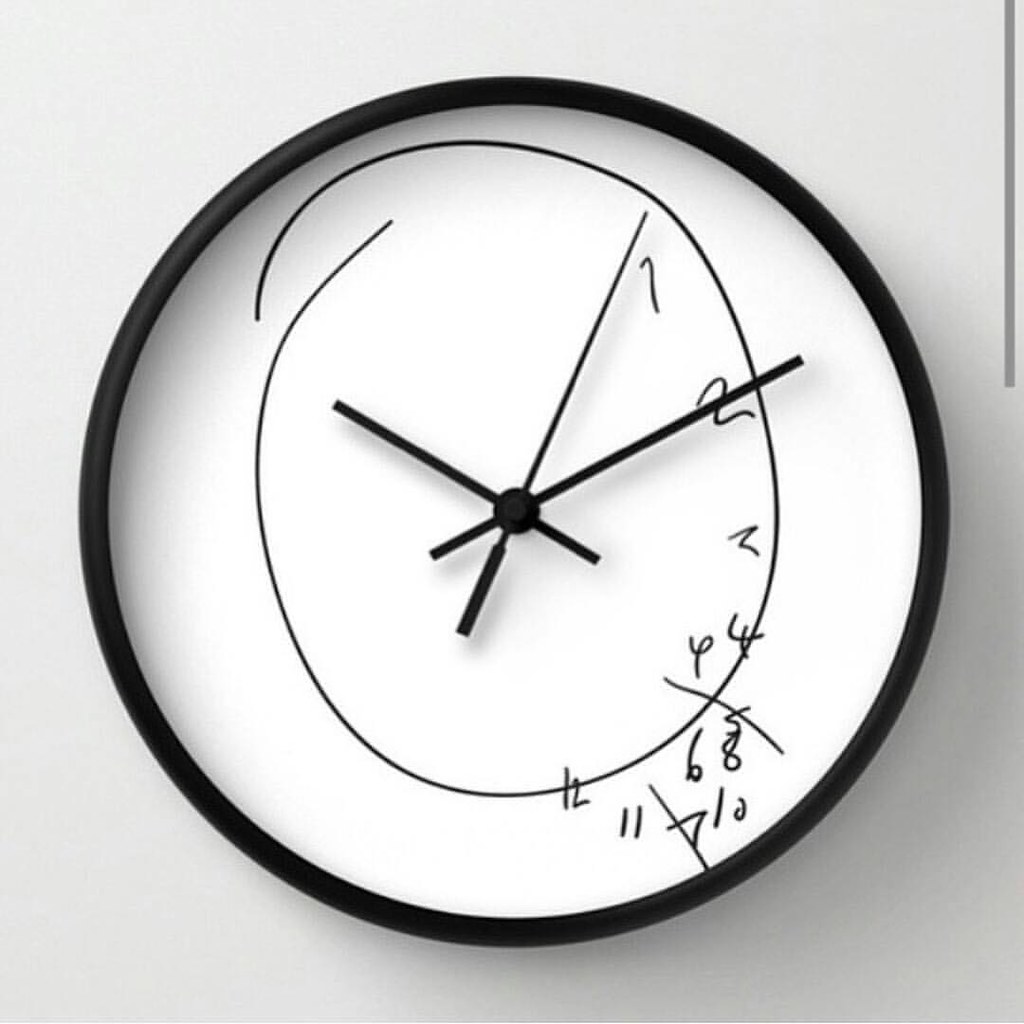The image features a digitally rendered, 3D-style clock mounted on a wall. The clock has a circular shape with a sleek black outer rim and a white face. The face is whimsically decorated with a haphazard black doodle, as if someone had drawn on it carelessly with a marker. Instead of the traditional clock numerals, the numbers appear jumbled and misplaced, giving the impression that they were drawn with closed eyes. From 1 to 12, the numbers are erratically positioned: with '1', '2', '3' in roughly the correct spots followed by a chaotic mix of '4', '6', '5', '6', '12', '11', '7', '10'. 

The clock hands include a prominent hour hand and a slightly longer minute hand. Also present is an unusually elongated third hand, likely representing the seconds. Based on the positions of the hands, the clock shows a time of about 10:10. 

A subtle shadow is cast to the bottom right of the image, adding a bit of depth. Additionally, there is a dark gray vertical stripe running from the top to the bottom, just along the right side of the white background, enhancing the overall visual context of the scene.